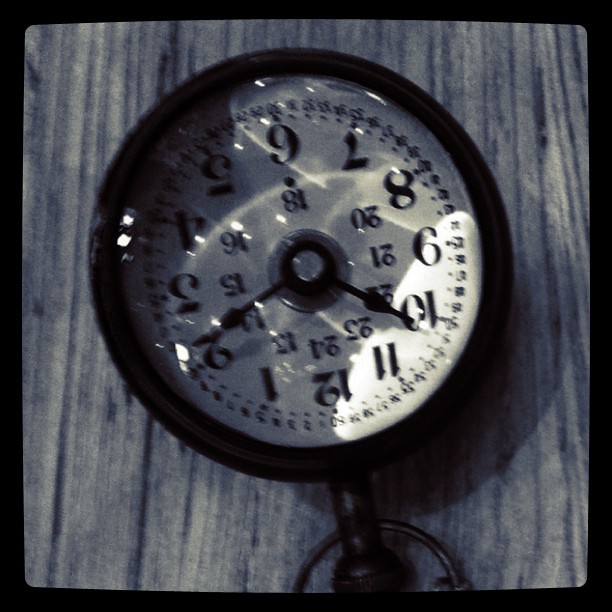This image captures a vintage pocket watch positioned so that the 12 o'clock mark is oriented towards the bottom of the photo. The watch is displayed against a square wooden background which contrasts with the black border of the photograph. The watch face itself is an elegant blend of white and pearl, featuring traditional black numerals. It indicates not only the hours but also the seconds with a separate track of numbers from 16 to 24 near the center. 

The central portion of the watch is silver, adorned by two black hands pointing out the hours and minutes, and an additional second hand. The light source creates a soft reflection, highlighting the right side of the watch while leaving the left side slightly shadowed. The pocket watch is encased in a dark, almost black metal, giving it a timeless appeal. 

At the base, the cylindrical stem, which transitions into a rounded edge, is oriented at the bottom of the image. This stem is accompanied by a circular metal ring, which is partly visible, resting just below it and slightly cut off by the edge of the picture.